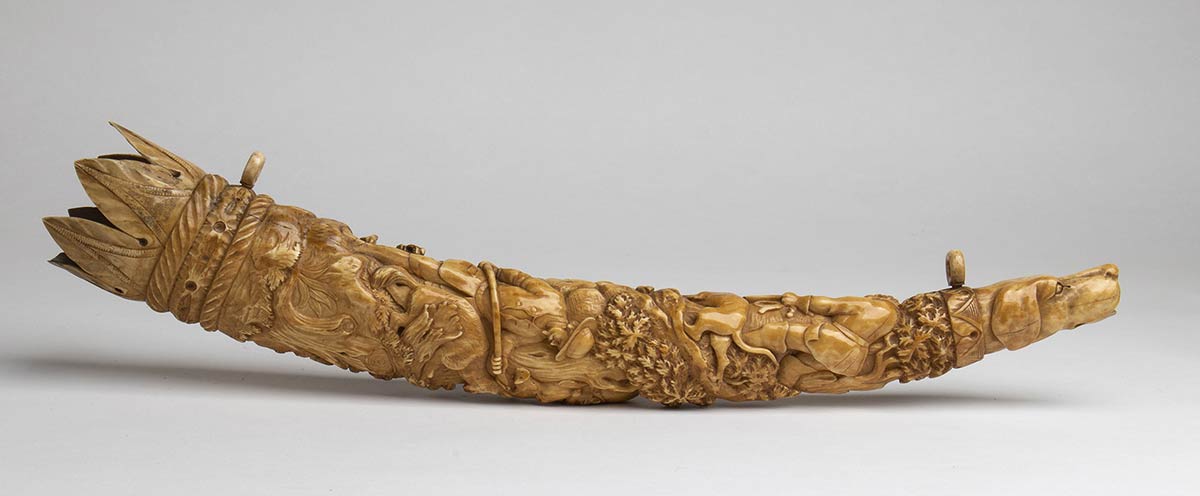The photograph showcases a meticulously carved ivory tusk, repurposed into a blow horn, set against a gray background. The upper half of the horn curves upward like a banana or a "U" shape, resting flat on the surface it is placed on. The horn’s dark sandy-colored surface features elaborate carvings that depict various cultural figures and scenes, telling a rich story of events. Notable details include a pointy area on the left tip, which broadens into a crown-like structure. Below the crown, the tusk displays three intricately woven rings carved into the ivory. Moving down the horn, the carvings transition into various scenes: a man holding a bloodhound under a tree, another man wielding a weapon attacking a boar, accompanied by another hound. The right end of the horn narrows and has been artistically shaped into the head of a dog. Two keyholes on either side of the top suggest that the horn can be strung up for display. The craftsmanship exudes depth, with the natural curvature and hollow form of the tusk preserved, reflecting an articulate and storied artistry.